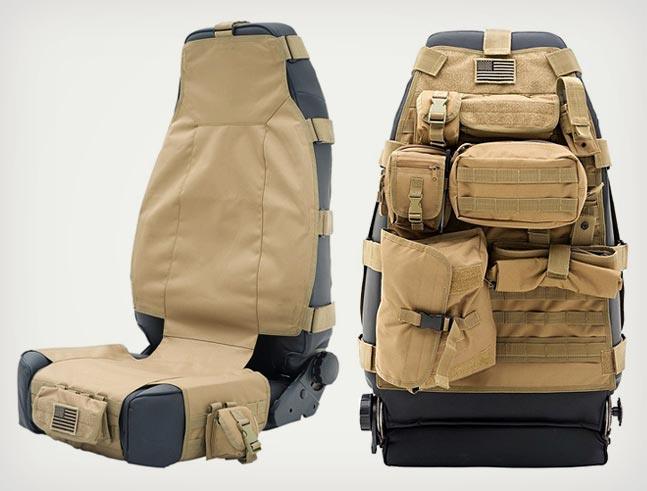This image features an innovative prototype of an automotive seat, specifically designed for standard driver and passenger seating in vehicles. The seat is upholstered in a light sand-colored material, giving it a sleek and refined appearance. The front portion, where the occupant sits, is secured with multiple straps—four on each side and an additional strap at the top, ensuring a firm and snug fit. 

A small rectangular section of sand-colored fabric connects the seat cushion to the front panel, which is also wrapped in the same sandy material. The fabric extends beneath the cushion, likely fastening with buckles or similar hardware. For added convenience, there are pouches strategically placed: one on the side of the seat and another at the front edge where the backs of the occupant’s legs would rest.

The back of the seat, visible from the rear seating area, is equipped with an array of practical pouches. These pouches vary in size and are abundantly spread across the backrest, providing ample storage for personal items and accessories. This innovative design maximizes storage space and enhances organizational efficiency within the vehicle.